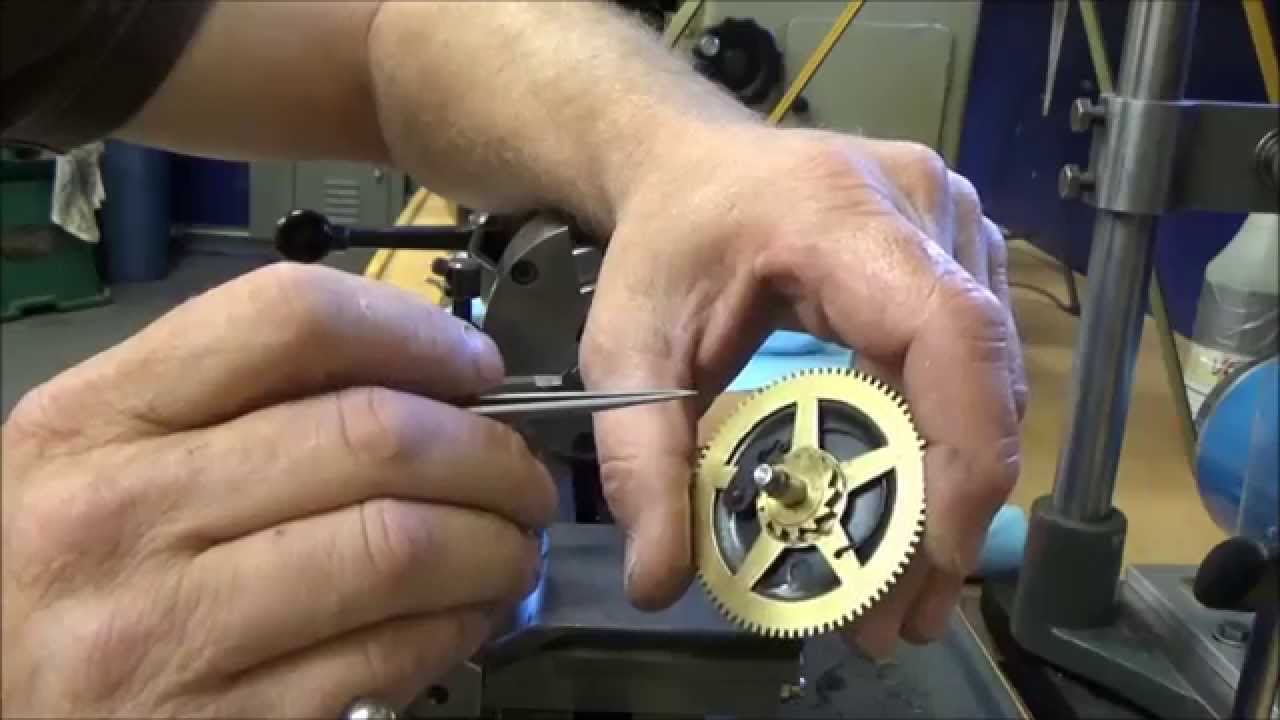In the image, a white man is meticulously working on a gold or bronze gear in what seems to be a well-lit workshop or factory setting. His left hand securely holds the gear, which measures about two inches in diameter and features numerous teeth for attachment to another mechanism. The gear also has a smaller, intricately designed cog in its center. In his right hand, he wields a tool or tweezers, poised to make precise adjustments to the gear. The man's arms are notably hairy, adorned with fine, light-colored hairs. His workspace includes a vice for stability and various tools. The background reveals tall, grey lockers and a green stool, reinforcing the industrial atmosphere. The lighting accentuates the metallic sheen of the gear, highlighting the man's focused effort to repair or fine-tune it.